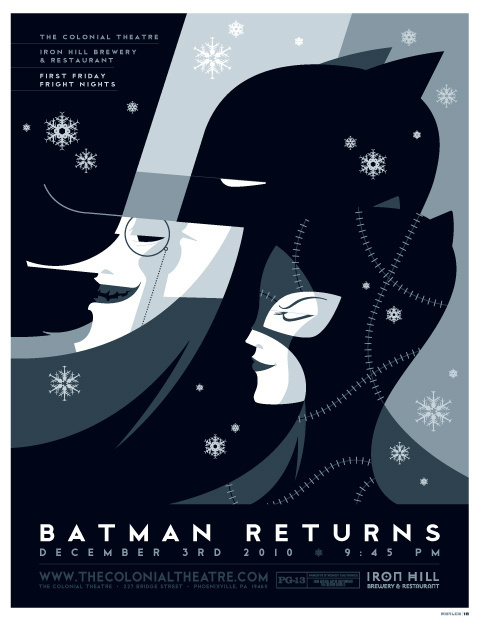This poster features an Art Deco-inspired illustration in shades of white, black, and grey. The artwork prominently displays the characters of Batman, Penguin, and Catwoman, the latter reminiscent of Michelle Pfeiffer's iconic stitched suit from the movie "Batman Returns." Surrounding the characters are delicate white snowflakes, adding a wintery touch.

In the top left corner, small white text announces the Colonial Theater and Iron Hill Brewery and Restaurant's event: "First Friday Fright Nights." Below the central illustration, a black bar with large white text boldly reads "Batman Returns," specifying the movie title. Beneath this, smaller grey text provides the event details: December 3rd, 2010, at 9:45 PM. The film is rated PG-13.

The event took place at the Colonial Theater located on Bridge Street in Phoenixville, Pennsylvania, and it was held approximately 14 years ago. Additional details, including the theater's website, www.thecolonialtheater.com, are also mentioned. This special presentation of "Batman Returns" was sponsored by Iron Hill Brewery and Restaurant, making it a notable community event.